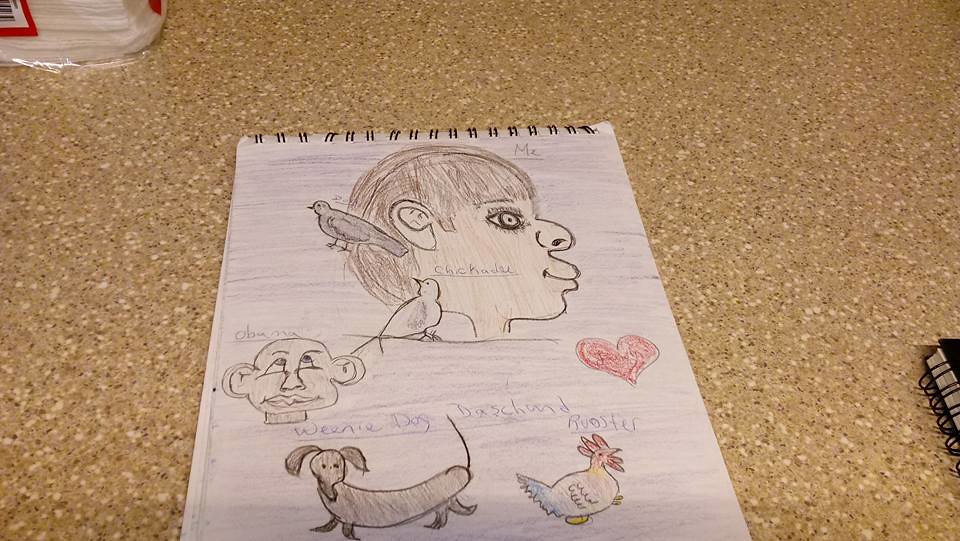A left-to-right horizontal photograph captured from a slightly downward angle, offering a partial view of the background context within an indoor setting. The image prominently displays a simple countertop with a mottled pattern of tans, beiges, and small brown dots. Positioned in the lower right corner is a black notebook with a black spiral binding. Toward the upper left, there is an item wrapped in plastic featuring a visible barcode. The focal point of the image is a hand-drawn illustration on another spiral-bound notebook, depicting a person's face, a heart, a chicken, a dog, and a figure resembling a man with exaggerated ears, all vividly colored in.